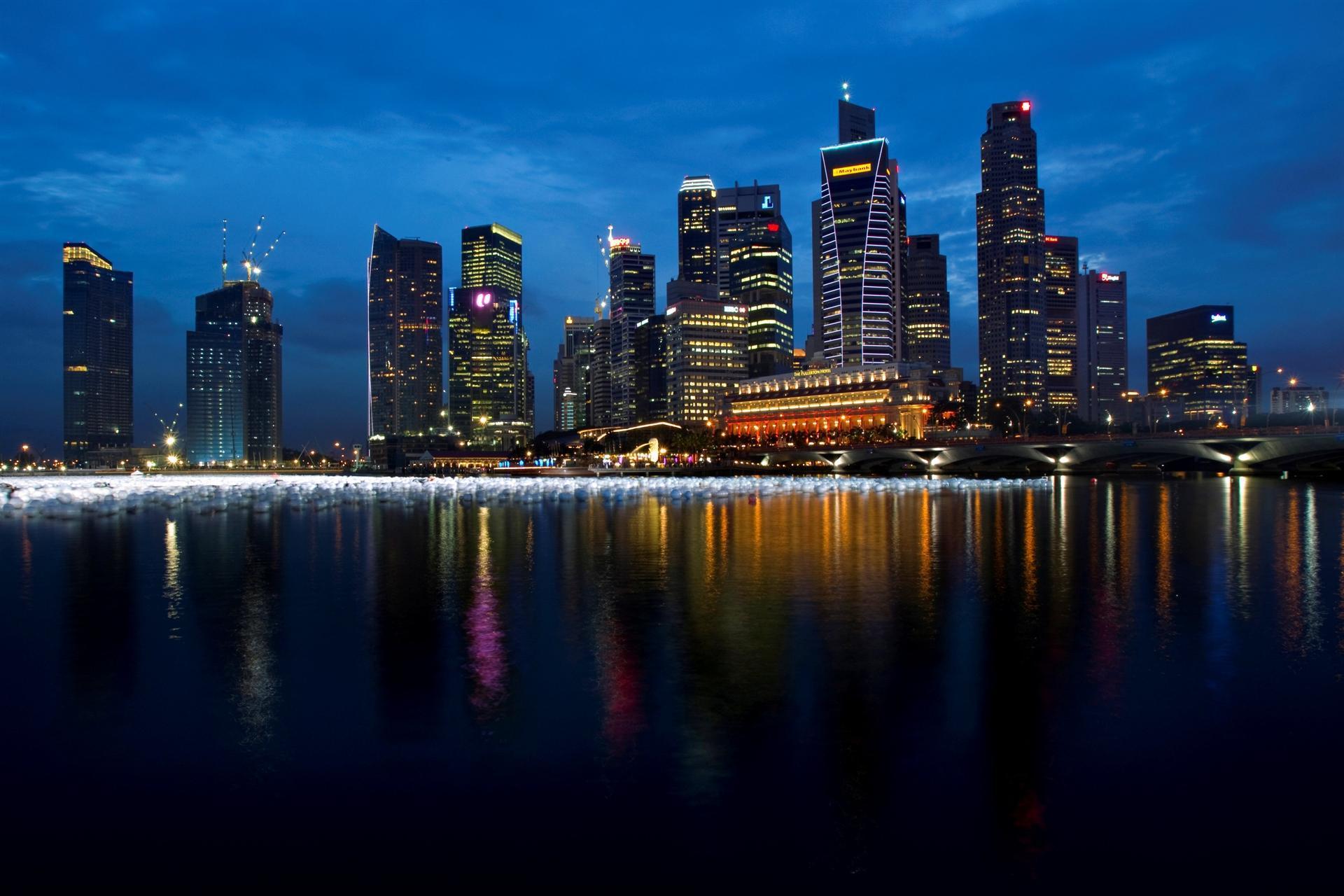In this captivating nighttime cityscape, a major metropolis is depicted under a dark, stormy-looking sky studded with heavy, gray clouds. The skyline is adorned with numerous towering skyscrapers, their windows aglow with vibrant yellow hues and adorned with various colored lights—white, pink, orange, and red—visible from the land and across a body of water. This water, occupying the bottom half of the image, is a deep, almost black blue, reflecting the myriad lights from the buildings and capturing the dynamic essence of the urban landscape. The water also features ripples and waves that break towards the shore, further enhancing the dramatic effect of the scene. A bridge spans the middle portion of the image, connecting the two sides of the city and adding architectural interest to the composite view. The combination of the lively reflections, the illuminated windows, and the dark, cloud-filled sky creates a splendid contrast, offering a vivid portrayal of a bustling city at twilight.